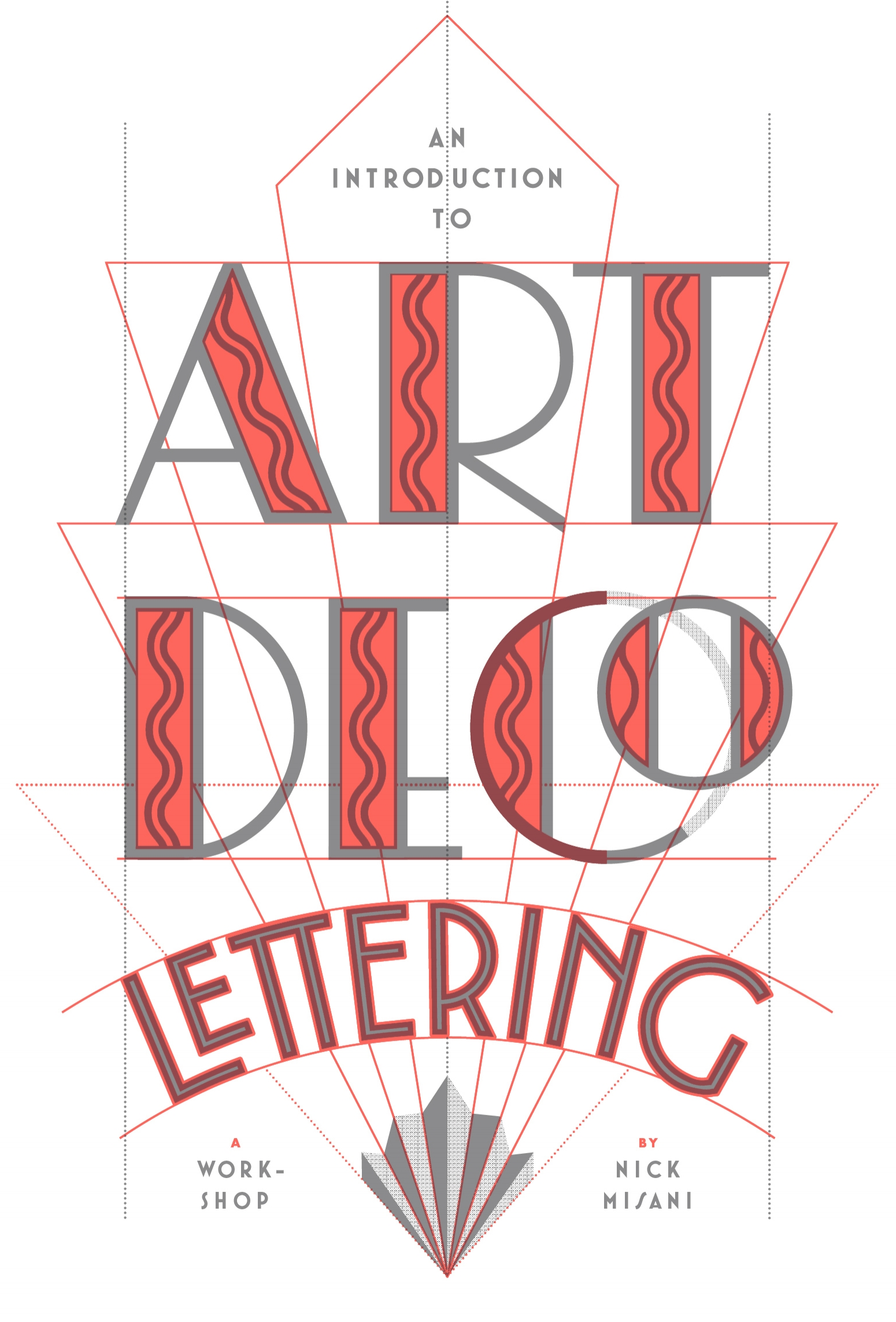The image is a digital advertisement on a white background promoting a workshop on Art Deco lettering. At the top, in small uppercase gray font, it reads "An Introduction to." Below this, in large artistic gray letters with a bold red outline, it says "Art Deco." This prominent text is surrounded by intricate red and blue lines, shaped into an upside-down V at the top, transitioning into fan-like designs and layered triangles as they move downwards. The word "Lettering," also in bold gray with a red outline, appears beneath "Art Deco" and is artistically curved. On the bottom left side, the image features "A Workshop" in red and gray font, with "By Nick Misani" written to the right, the latter in small red font. The overall layout combines structural elements with flowing, wavy lines, creating a visually engaging and detailed presentation for this instructional event.